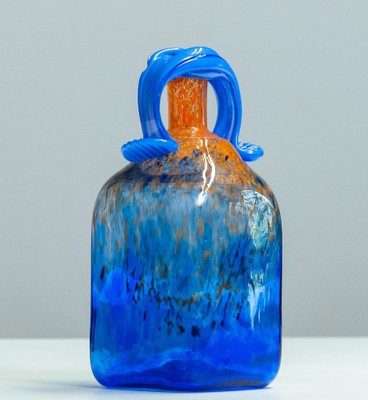The image showcases a captivating artist's interpretation of a jug crafted from glass, featuring an unconventional handle design. The handle, resembling twisted taffy, arches gracefully over and above the spout, presenting an almost edible appearance due to its pure and intricate twists. The jug itself is a kaleidoscope of colors, seamlessly blending from aqua blue, aquamarine, and aqua green to blue and royal blue, culminating in a vibrant orange that speckles the spout. A brilliant opening is subtly integrated within the twist of the handle, barely visible yet hinting at its separation from the spout. The background is a light gray, which adds a touch of sophistication, while the jug rests elegantly on a pristine white surface.